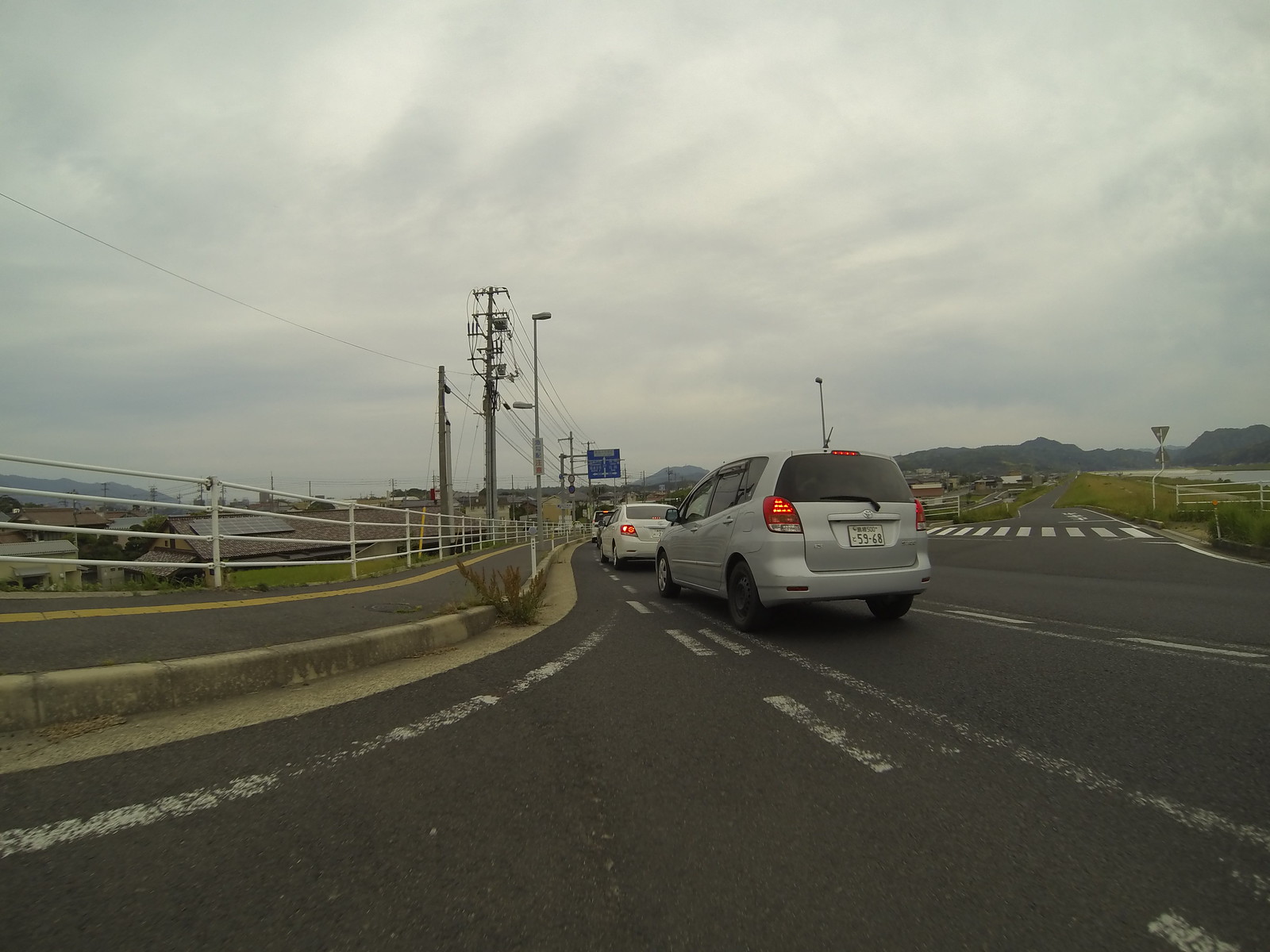The image depicts a bustling road scene with several cars, including a white car and a silver van, stopped in the left lane with their brake lights illuminated. The road forks off to the right where a clearly marked pedestrian walkway with white stripes is visible. This secondary road stretches into the distance, flanked by green grassy fields on both sides, leading toward a tranquil body of water with majestic mountains rising in the background. The overcast sky casts a gray hue over the scene, complemented by the white, cloudy atmosphere. The main road is bordered by a concrete curb and a metal railing fence on the left, with power lines and streetlights adding an urban touch. In the distance, an indistinct green highway sign can be seen, though its text is not legible. Various elements such as telephone wires, safety railings, and vibrant vegetation pepper the landscape, and the presence of yellow lines along the sidewalk suggests an area designed with safety in mind, potentially indicating an Asian setting.